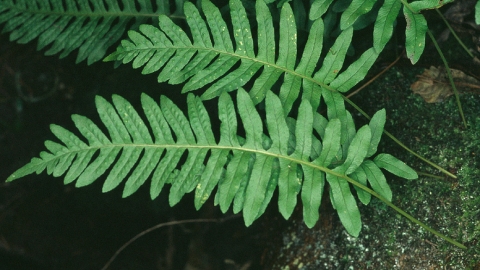The photograph captures a cluster of ferns, prominently featuring two long, narrow leaves with thin, pointed leaflets, nestled on a moss-covered rock. The ferns, which appear vibrant and healthy in their medium green hue, are dotted with dew drops, adding a touch of freshness. The rock surface hosts a mix of moss and a single dead leaf, enhancing the natural setting. The background is dark, providing a stark contrast that accentuates the greenery. Small twigs and a few other ferns partially visible in the corners, along with hints of other plants, complete the scene. The overall colors in the image are predominantly green, gray, black, and white.